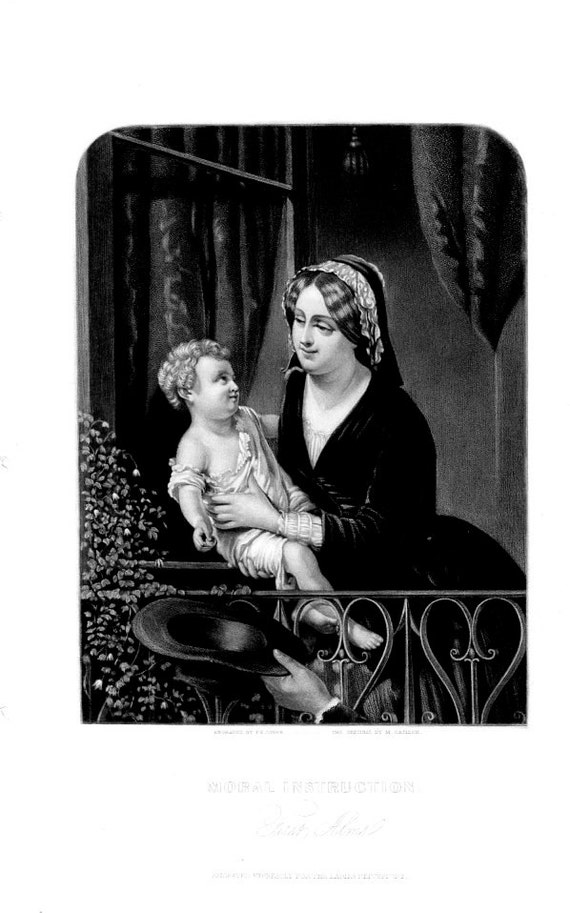This detailed black-and-white painting captures an intimate moment between a mother and her toddler on a balcony. The woman, with her short, dark hair tucked under a patterned cloth headpiece, is attired in a black dress with a white frilled shirt underneath. She leans forward affectionately, gazing at her son with a slight smirk. The toddler, with curly hair that barely reaches his ears, is clad in a white outfit that loosely slips down his left shoulder. He returns his mother's gaze lovingly, his delicate fingers clutching her arm. 

The backdrop features an ornate wrought iron railing adorned with heart-shaped designs, indicating they are on a balcony. To the left, vines creep up the side of a home, adding a touch of nature to the scene. The large window behind them has open curtains and a chandelier hanging above the woman's head, emphasizing the indoor-outdoor blend. Part of a man's outstretched hand with a top hat open is visible at the bottom right, hinting at another figure in the scene. This evocative artwork likely from the 1800s captures the tender bond between mother and child, surrounded by intricate details that enhance its vintage charm.